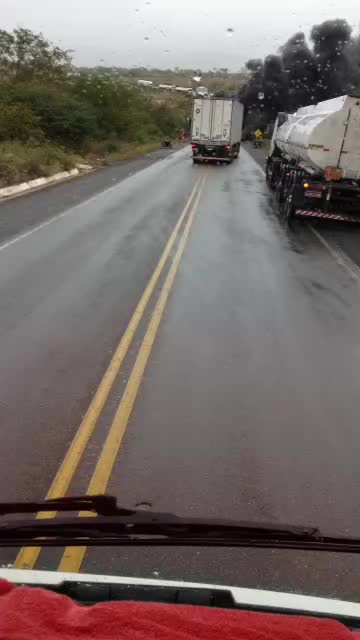This photograph, taken from inside a high-seated vehicle such as an RV or big rig, captures a rainy afternoon on a rural two-lane highway. The viewer's perspective includes a strip of the vehicle’s white hood, a visible windshield wiper, and a red towel resting on the dash replete with raindrops. The highway extends straight ahead and is flanked by mounds of trees with some appearing brown in the distance. A white tanker truck, with a black cab, is pulled onto the shoulder, while a white box-shaped semi-truck, with its brake lights illuminated, is overtaking it and crossing the double yellow lines to return to the proper lane. The gray, overcast sky and wet asphalt underscore the damp, dreary weather.